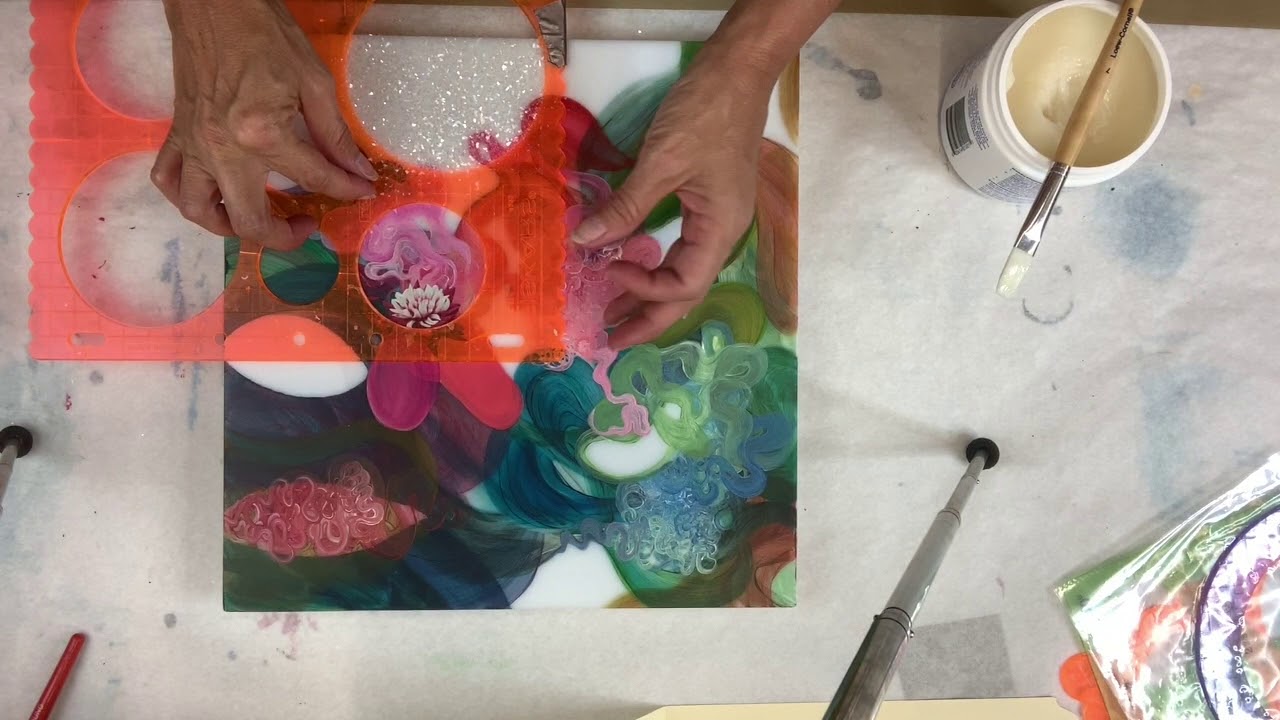In this bird's-eye view photograph, an artist is engrossed in creating a vibrant piece on a square canvas protected by a layer of white paper to keep the workspace clean. The artist's two hands, partially visible, are at work with a red plastic circular stencil, guiding the arrangement of intricate floral patterns and colorful spirals. The painting showcases a lively palette with swirls and splotches of green, blue, pink, purple, and red, creating a marbled effect. A jar of clear-ish gel, possibly glue or clear paint, rests on the right, capped with a paintbrush. Nearby, a plate with paper adorned in beautiful blue and purple tones adds to the artistic chaos. Additionally, a cell phone stand is visible, hinting at a recorded or livestreamed creative session, with some bright cellophane peeking out from the right.